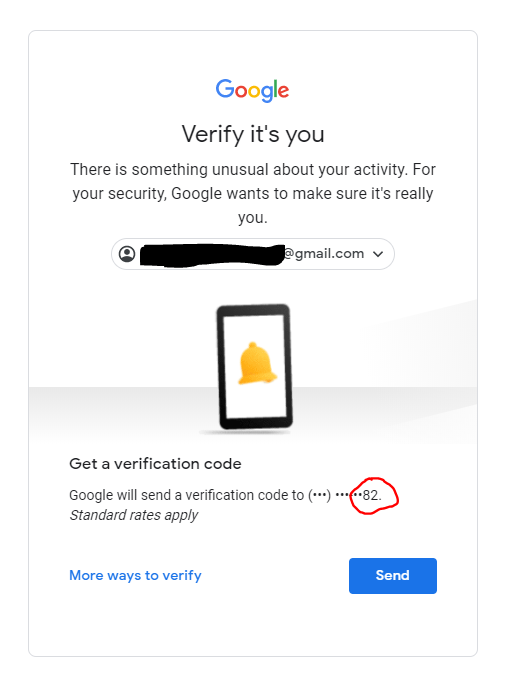The image appears to be a screenshot taken on a tablet, displaying a Google verification page. At the very top center of the page, the colorful Google logo is prominent; the capital 'G' is blue, the first 'o' is red, the second 'o' is yellow, the 'g' is blue, the 'l' is green, and the 'e' is red, slightly tilted. Just below the logo, centered and in bold black letters, the text reads "Verify it's you." 

Beneath this bold text, in regular black letters, is the message: "There is something unusual about your activity. For your security, Google wants to make sure it’s really you." Following this text, there is a long oval section with a blacked-out email address, revealing only the ending "@gmail.com."

Centered below the email address is an icon depicting a smartphone or tablet, outlined in blue with a white background, and featuring an orange alert bell. The screen transitions into a light gray faded area that instructs, "Get a verification code." It further explains, "Google will send a verification code to," with the phone number partially obscured, displaying only the last two digits "82" highlighted in red.

Below the phone number, in italicized font, the text "Standard rates apply" is displayed. At the very bottom of the page, there are two options: in blue text, "More ways to verify," and a blue rectangular button with "Send" in white lettering, indicating it is clickable.